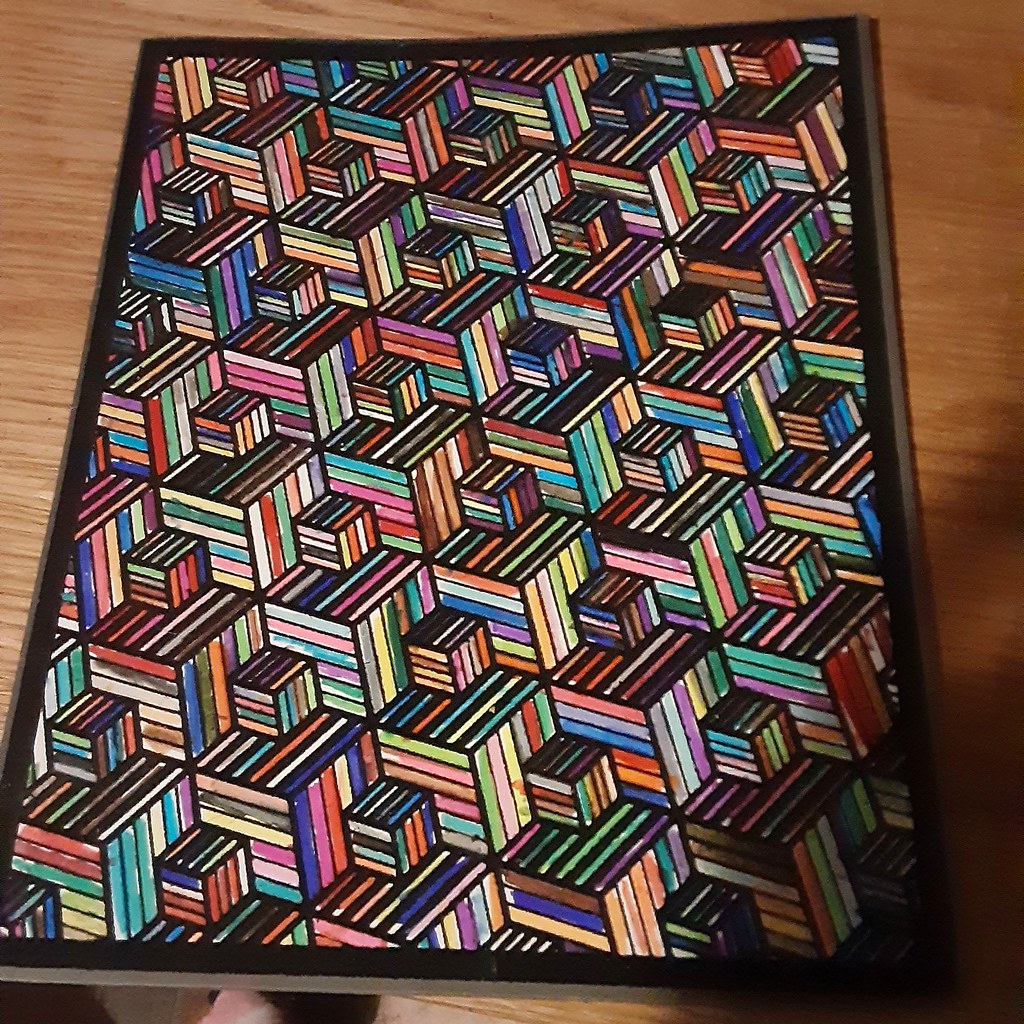This photograph captures a vibrant, geometric artwork, possibly a rug or a painting, displayed flat on a wooden table. The piece measures approximately 12 by 16 inches and is framed in brown. The artwork features a series of cubes in various sizes, with smaller cubes about one-quarter the size of the larger ones. These cubes are adorned with colorful stripes and outlined in black, showcasing a range of colors including purple, pink, green, yellow, red, gray, teal, and black. The arrangement resembles a tumbling blocks quilt pattern, with each smaller cube positioned at the intersection of two larger cubes, aligned directionally with matching stripes. The geometric arrangement of the stacked cubes extends from one end of the piece to the other, creating a visually striking and colorful display bordered in gray and black.